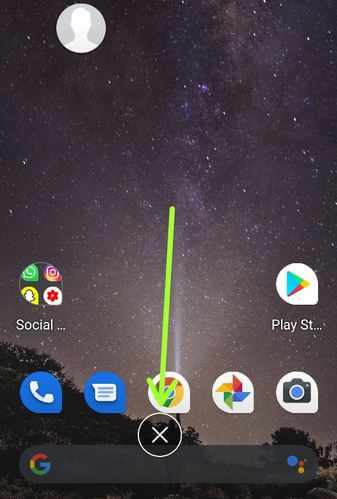The image captures the bottom two-thirds of a smartphone's home screen, possibly indicating a shorter screen. The background is a stunning night sky filled with stars and star clusters, transitioning near the bottom to silhouettes of tree tops and leaves. 

Towards the upper left corner, there's a profile icon displaying a white torso and head against a simple gray background within a circle. 

Below, there's a section dedicated to social apps, displayed as a series of grouped icons. To the right of this section, a uniquely shaped icon for the Play Store is visible. This icon is designed with a line across the bottom right and a vertical line on the right edge, resembling the simplistic shape of an 'A' or a tilted teardrop.

At the very bottom, there are quick-access icons for essential apps including phone, chat, Chrome, an unidentified pinwheel logo (possibly Google), and a camera. Beneath these icons is a close (X) button.

A prominent feature is a large green arrow extending from the middle of the constellation area, pointing directly down at the close (X) button encased in a circle.

Finally, below all other elements, there is a search field featuring a 'G' logo with a simple gray overlay.